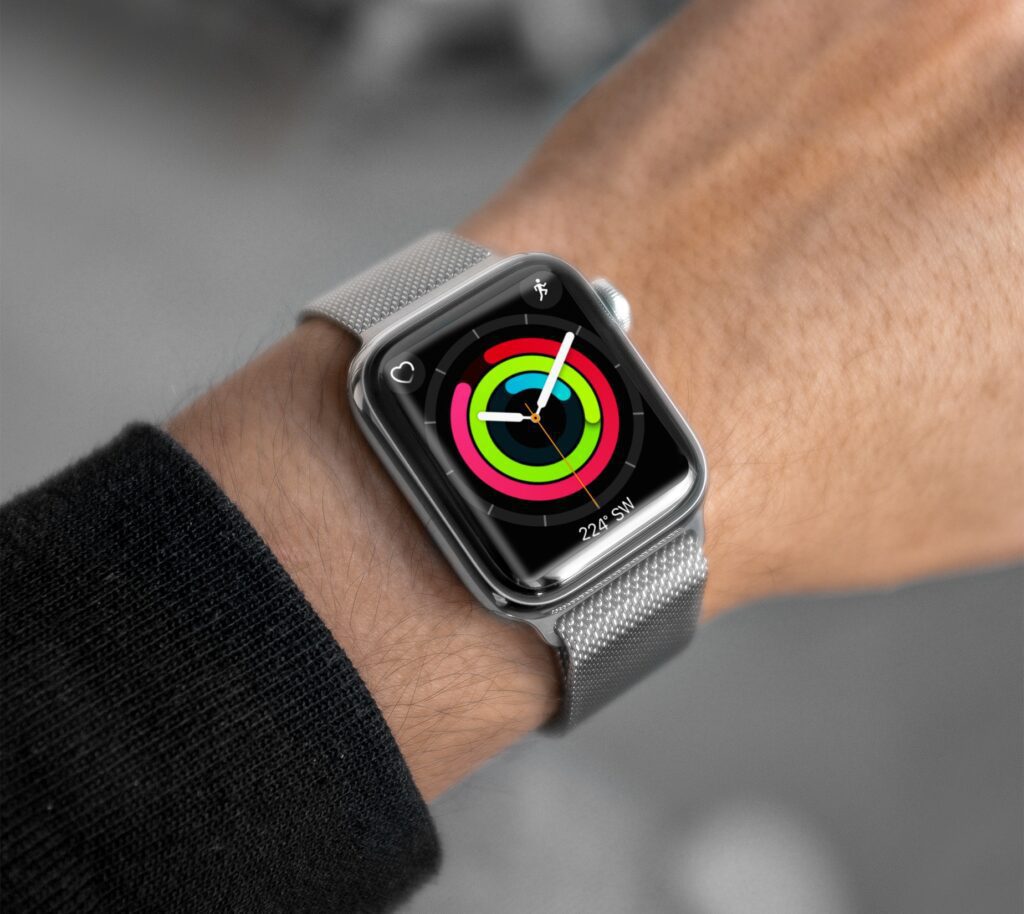The image captures a close-up view of an Apple Watch wrapped around a man's wrist, who has a tan skin complexion and is dressed in a dark, long-sleeve shirt. The Apple Watch features a metallic silver strap that complements its sleek and manly appearance. The black watch face prominently displays the time in an analog fashion, with three concentric activity circles in green, blue, and a gradient from red to pink, tracking the wearer's movement and calories. Additional icons, including a heart in the top left corner, a running person in the top right corner, and a compass marker at the bottom center reading "224° Southwest," are clearly visible. The overall image is in color and well-lit with natural lighting, while the background is grayed out and out of focus, ensuring that the Apple Watch remains the focal point of the photograph.